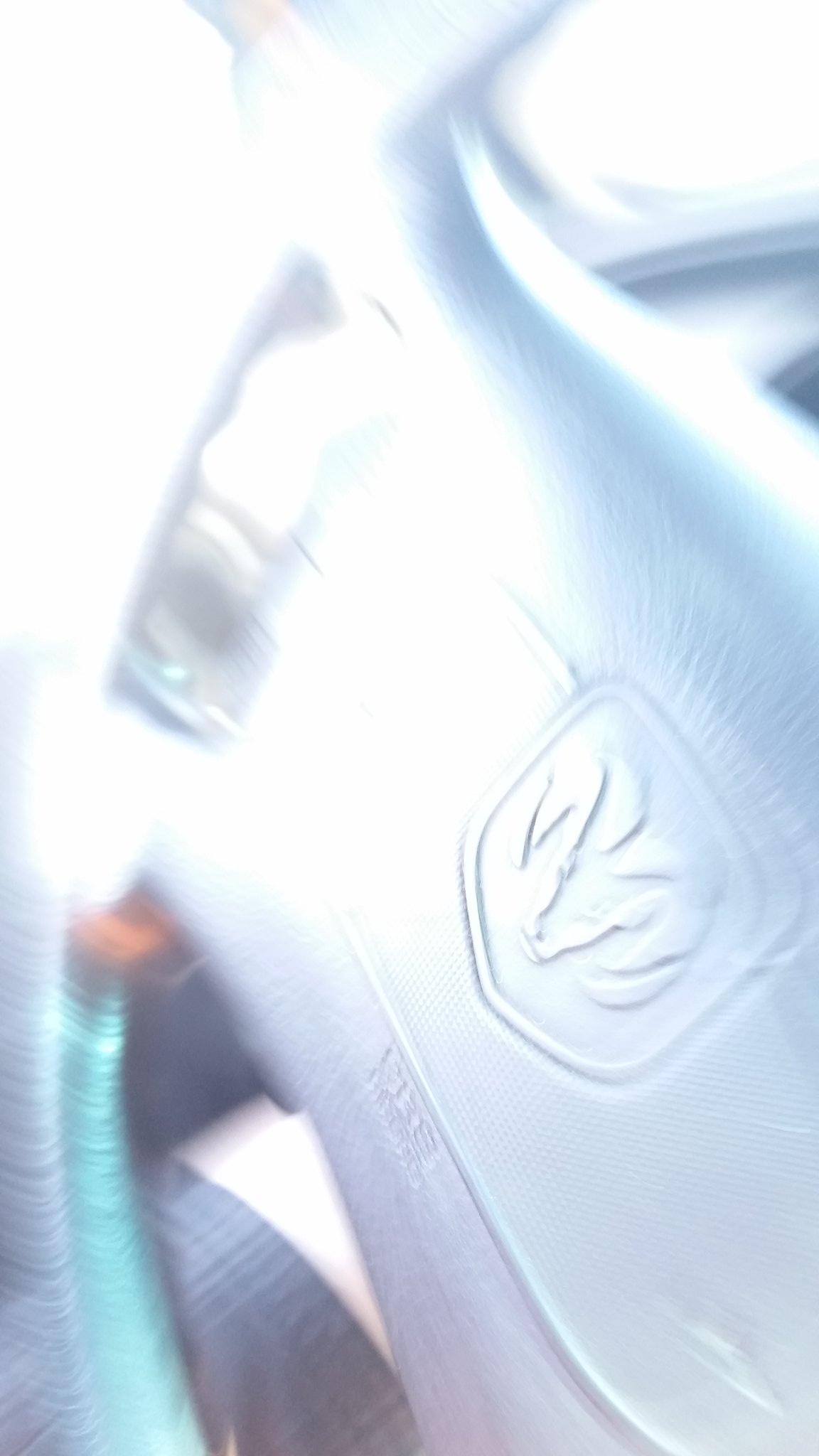In this blurred and low-resolution image, the photograph appears heavily filtered, giving it an extremely light and washed-out appearance. The focal point of the image is a silvery gray object, which seems to be some type of container or bag. The container is a light gray color with an opening at the lower left, oriented vertically. Inside this opening, a smaller object can be seen, featuring white and blue hues, though its exact nature is indeterminate. Notably, in the upper right corner of the container, there is a distinct label that appears to have an engraved outline of a ram. The faint details add a mysterious and almost ethereal quality to the photograph, leaving much to the viewer's imagination.